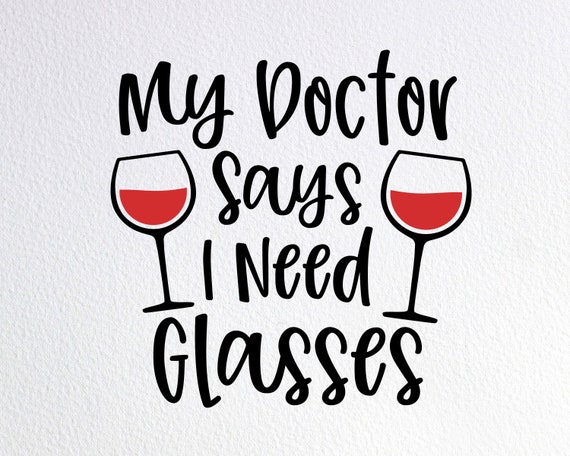The image is a detailed drawing presented on what appears to be textured light gray paper, resembling a poster or a painting. Centrally positioned in mildly cursive black text spanning four lines, the phrase "My doctor says I need glasses" catches the eye. On both the left and right sides of this humorous statement, there are black outline drawings of two wine glasses, each filled halfway with a rich red liquid, representing red wine. The wine glasses, drawn symmetrically around the text, emphasize the clever play on words, substituting wine glasses for eyeglasses to create a lighthearted, comedic effect. The entire composition sits within a square frame, enhancing its balanced and aesthetically pleasing layout.